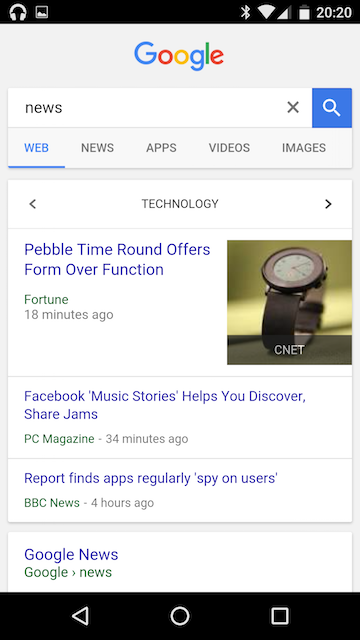The screenshot captures a Google search results page on someone's phone. At the top of the screen, a black notification bar displays white headphone icons on the left, indicating the user has headphones connected. The time displayed is "2020," presented in military format.

Below this, a light gray background prominently features the Google logo in its signature colors: blue, red, yellow, blue, green, and red, spelling "Google." Beneath the logo, a navigation bar has a white box with the word "News" in black, flanked by a gray "X" on the right and a blue box with a white magnifying glass icon.

The page shows five tabs for different search categories. The first tab, labeled "Web," is highlighted in blue with a blue underline, indicating the current active section. The other tabs listed are "News," "Apps," "Videos," and "Images."

Further down, a white search box displays the word "Technology" in black text, accompanied by left and right arrows for scrolling. Below this, a thin gray line separates the search box from the search results.

The search results show a series of headlines:

1. "Pebble Time Round offers form over function" (in blue), attributed to Fortune (in green), posted 18 minutes ago (in black).
2. "Facebook Music Stories help you discover and share jams" (in blue), attributed to PC Magazine (in green), posted 34 minutes ago (in black).
3. "Report finds apps regularly spy on users" (in blue), attributed to BBC News (in green), posted 4 hours ago (in black).

At the bottom of the screenshot, "Google News" is displayed in blue and red text.